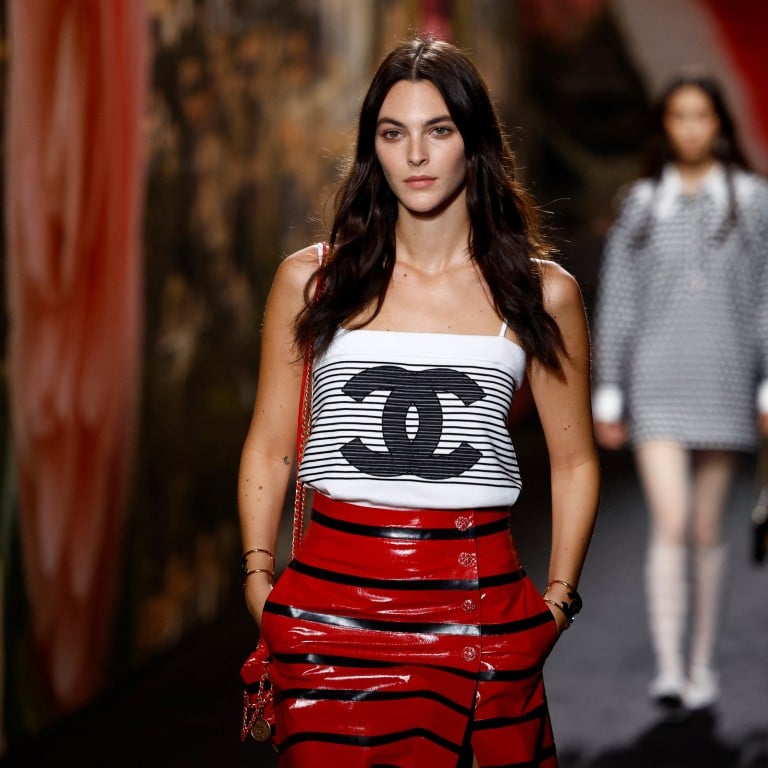In this image, two women are captured on a fashion runway. The focus is on the model in the foreground, who exudes confidence with her chest-length, wavy black hair parted in the middle. She is dressed in a striking ensemble featuring a white sleeveless top adorned with several black horizontal straps and a bold, overlapping double C logo, reminiscent of Chanel, emblazoned across the chest. Her top is paired with a shiny, possibly leather red skirt that is accented with black horizontal stripes, giving it a dynamic and edgy appearance. She appears to be holding a red purse over her shoulder and has her hands placed in the skirt's pockets, adding to her poised demeanor.

In the background, slightly out of focus, another model with long black hair is visible. She is dressed in a mini dress with a white collar and white cuffs, featuring a black and gray pattern. She also sports white knee-high socks and white boots, contributing to a cohesive monochromatic look. The runway floor is gray, and the backdrop is a burst of artistic colors - red, yellow, and black - which may contain an indistinct picture.

Despite the blurred details in the surroundings, the models stand out prominently against the artistic and vibrant setting, encapsulating the essence of a high-energy fashion show.